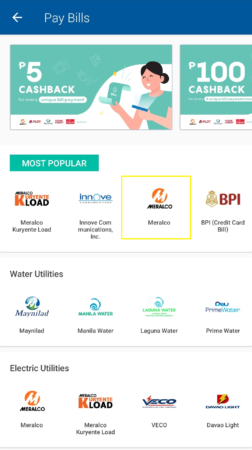The image features a user interface for a financial service platform centered around bill payments. In the upper left corner, there is a "Pay Bills" option highlighted on a blue strip with white font accompanied by a left arrow icon. Directly below this, text reads "P5 Cash Back." Unfortunately, some smaller font details and icons in this section are too blurry to decipher.

In the center of the image is a green rectangle containing a cartoon illustration of a woman with dark hair styled in a low bun. She appears to be holding a bill or money in her hand. To the right of this image, text reads "P100 Cash Back." Below this, there is another text block where partial words can be seen, likely including phrases like "most popular k-load in OVA" and "Mercado."

Further below, there are several service categories listed, though many are difficult to read due to poor resolution. Among the discernible categories are "VIP Credit Card," "VIP Water Utilities," "MAYNILAD," and possibly "Prime Water" and "Electric Utilities." Despite the low image quality, the overall message seems to promote cash back incentives for paying bills through this platform.